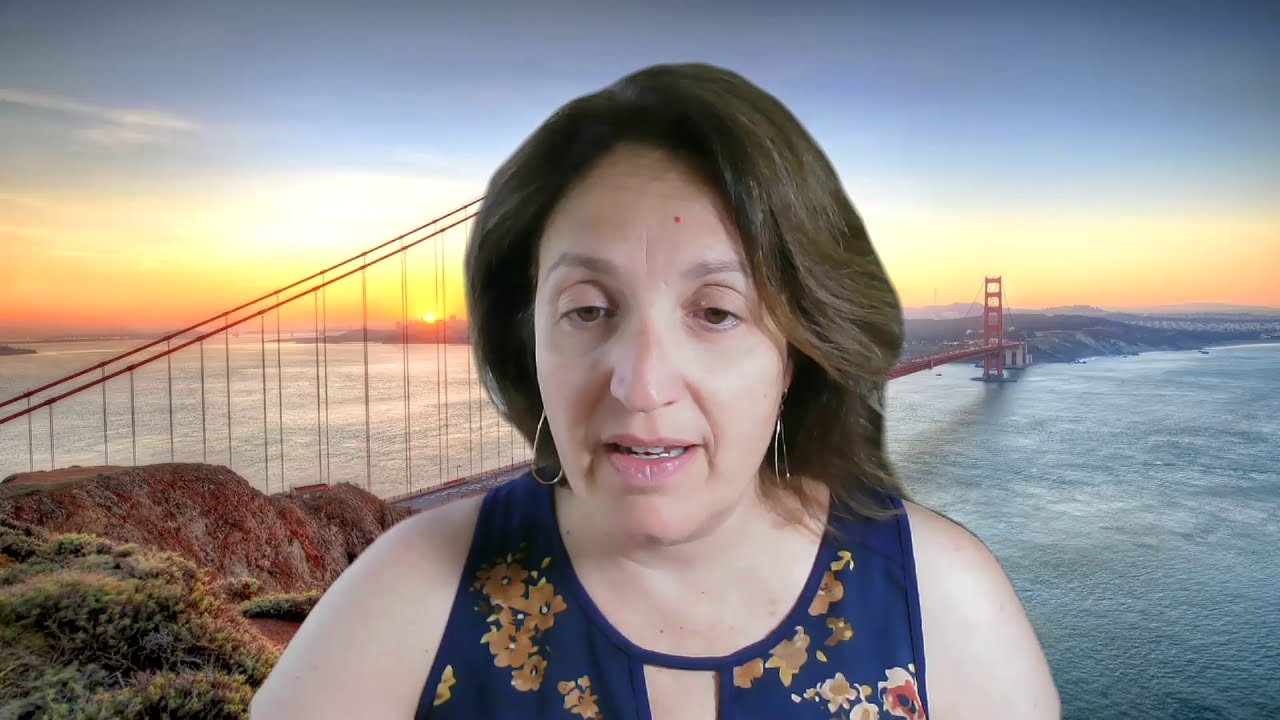In this horizontal rectangular image, a woman is prominently featured at the center. She appears to be in her 40s with slightly wavy, shoulder-length brown hair and heavy eyelids. She is gazing slightly down to her left, her body facing forward. Her lips, adorned with light pink lipstick, are parted as if she is speaking, revealing her teeth. Large gold hoop earrings complement her look, along with a sleeveless navy blue shirt featuring a gold floral pattern and a cutout in the chest area.

Behind her stretches a serene body of water, likely the ocean, as the Golden Gate Bridge spans the background. The sky above is a gradient of blue with the sun setting, casting hues of orange, pink, and yellow across the clouds. The sun itself is a small orange ball peeking through the clouds. The grass and rocky area can be seen to her left, adding depth and texture to the scene. This vivid outdoor setting, bathed in the colors of sunset, captures a tranquil moment amidst the natural and man-made wonders.